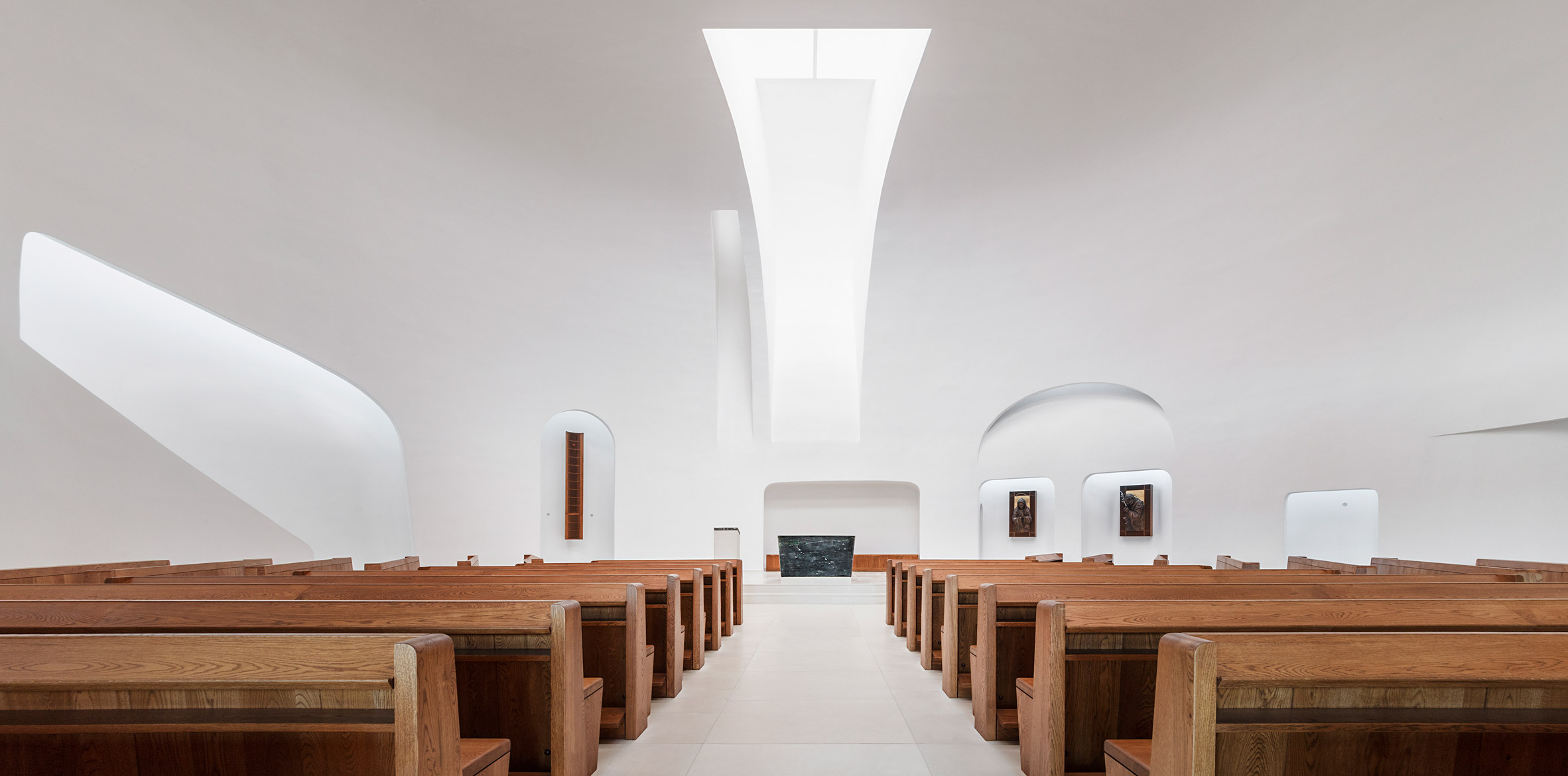This image depicts the interior of a modern church with a stark white architectural style. The spacious room features approximately ten to twelve rows of wide wooden pews, evenly divided with six on the left and six on the right, facing towards the front. Notably, two additional rows of pews are situated in a semi-circular arrangement, creating a shell-like formation. A clear central aisle separates the rows, leading up to a dark granite altar at the far end of the room. The pristine white tile floor complements the uniformly white walls, which are adorned with a couple of pieces of artwork on the right-hand side. The church is illuminated by a skylight, casting additional light that reflects off the left side of the room, enhancing its clean and pure ambiance. There are no people, animals, writing, mechanical objects, or motor vehicles visible in this photograph, emphasizing the serene and uncluttered design of the modern place of worship.